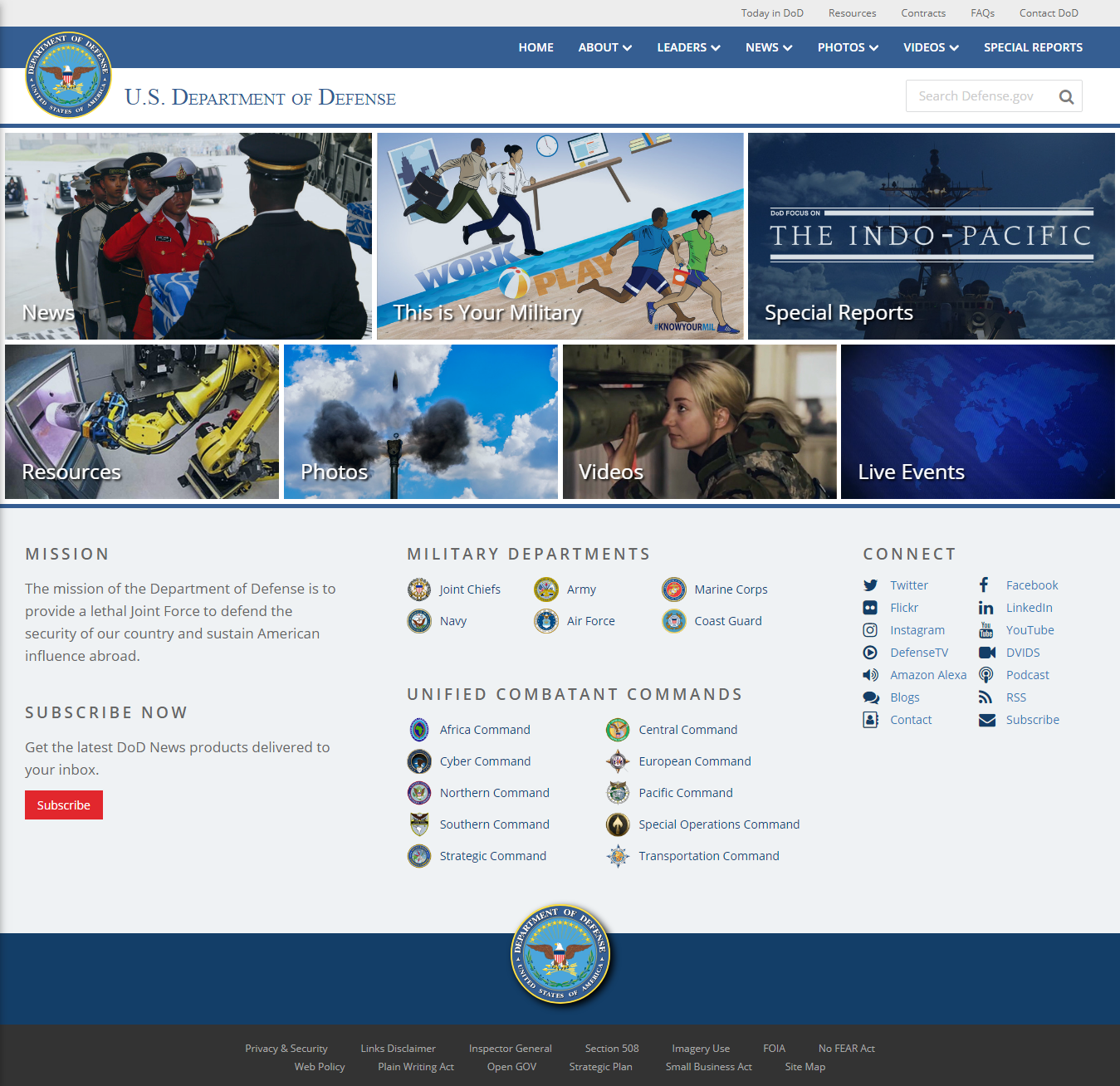This image depicts a webpage from the U.S. Department of Defense. The official emblem featuring an eagle encircled by text is prominently displayed. The navigation menu on the upper section of the page contains the following options: "Home," "About" (with a drop-down menu), "Leaders" (with a drop-down menu), "News" (with a drop-down menu), "Photos," "Videos," and "Special Reports." Beneath this menu, there is a search bar labeled "Search Defense Government."

At the top of the webpage, additional navigation options are listed: "Today in DoD," "Resources," "Contacts," "Facts," and "Contact DoD." The central part of the page features various images, including service members saluting and standing in formation. Under the "News" section, there's a headline that reads "This is Your Military," accompanied by cartoon-drawn characters. There's also a mention of the "Indian Pacific" in the context of special reports.

Further down, in a highlighted section with a white background, there are additional elements, such as "Missions" and a red "Subscribe Now" button for users to subscribe. The "Military Departments" section displays six icons representing different branches, including the Coast Guard. Additionally, the "Unified Combatant Commands" and a section for "Connect" with various social media icons are present, offering ways for users to engage with the Department of Defense online.